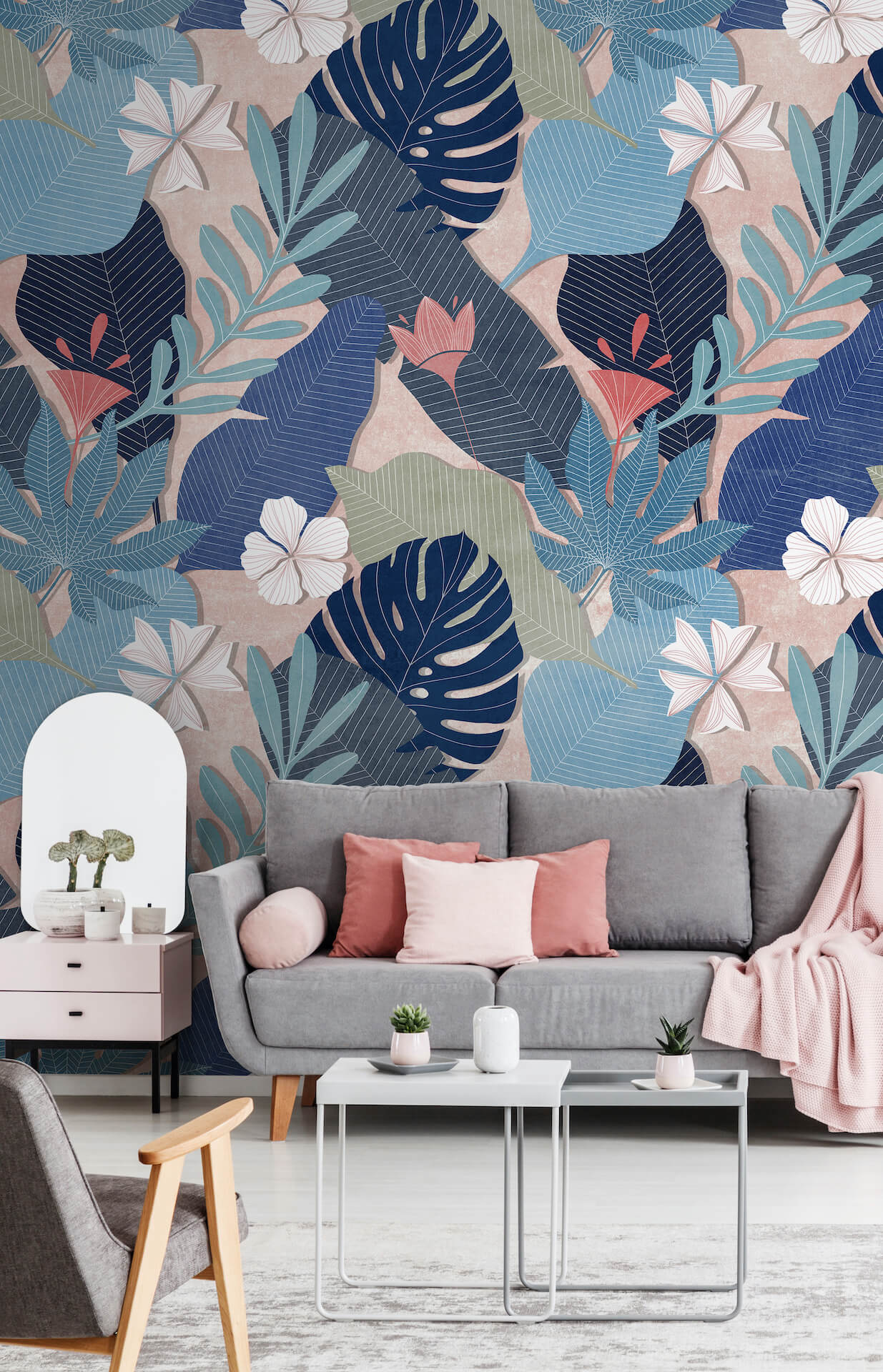The image depicts an eclectic and vividly decorated living room, highlighted by a bold floral wallpaper that gives the impression of being three-dimensional, with its array of flowers and fern-like leaves in a riot of colors including orange, reddish, blue, green, pink, and white. Dominating the right side is a gray couch adorned with coral, light pink, and light-colored pillows, complemented by a light pink throw blanket. In front of the couch stands a white coffee table hosting various white potted plants, possibly an aloe vera or cocktail plant, adding a touch of nature to the setting. To the left, there's a light pink side table also holding a potted plant beneath a mirror that reflects part of the greenery. A matching gray chair with a wooden frame sits across from the couch, and a gray rug grounds the seating area. Additionally, the bottom left corner reveals a black seat with wooden armrests, and between it and the couch, there are two square tables in light blue and gray, each adorned with small potted plants. The overall scene is cohesive yet lively, emphasizing a mix of colors and textures for a vibrant interior décor.